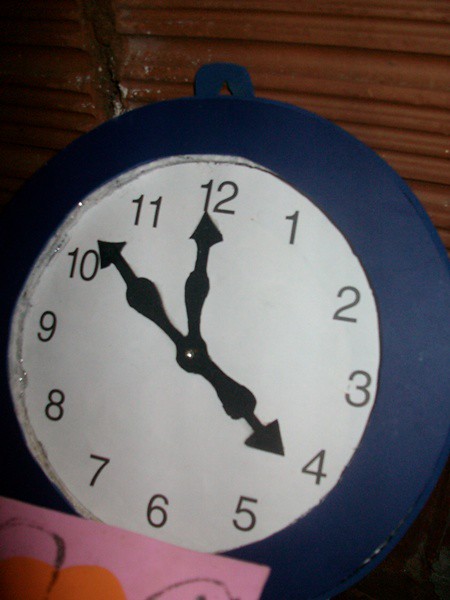This up-close photograph prominently features a round analog clock. The upper part of the image showcases a wood grain background in varying shades of brown, with visible horizontal lines. The clock itself has a thick, navy blue outer ring with a white face. Black numbers marking 1 through 12 accurately encircle the face. The hour, minute, and second hands—all black and ending in arrowheads—are distinctly visible; the hour hand points to 12, the minute hand between 4 and 5, and the second hand between 10 and 11. At the top of the clock, there's a handle hole. 

In the lower left-hand corner, partially obscuring the clock, is a piece of pink construction paper with some black and red paint and a hint of orange, possibly part of a sticker. The pink paper appears to lean against the brown background, adding a slight splash of color to the image. An additional detail is that the clock seems to be made from a felt-like material, giving it a textured appearance.